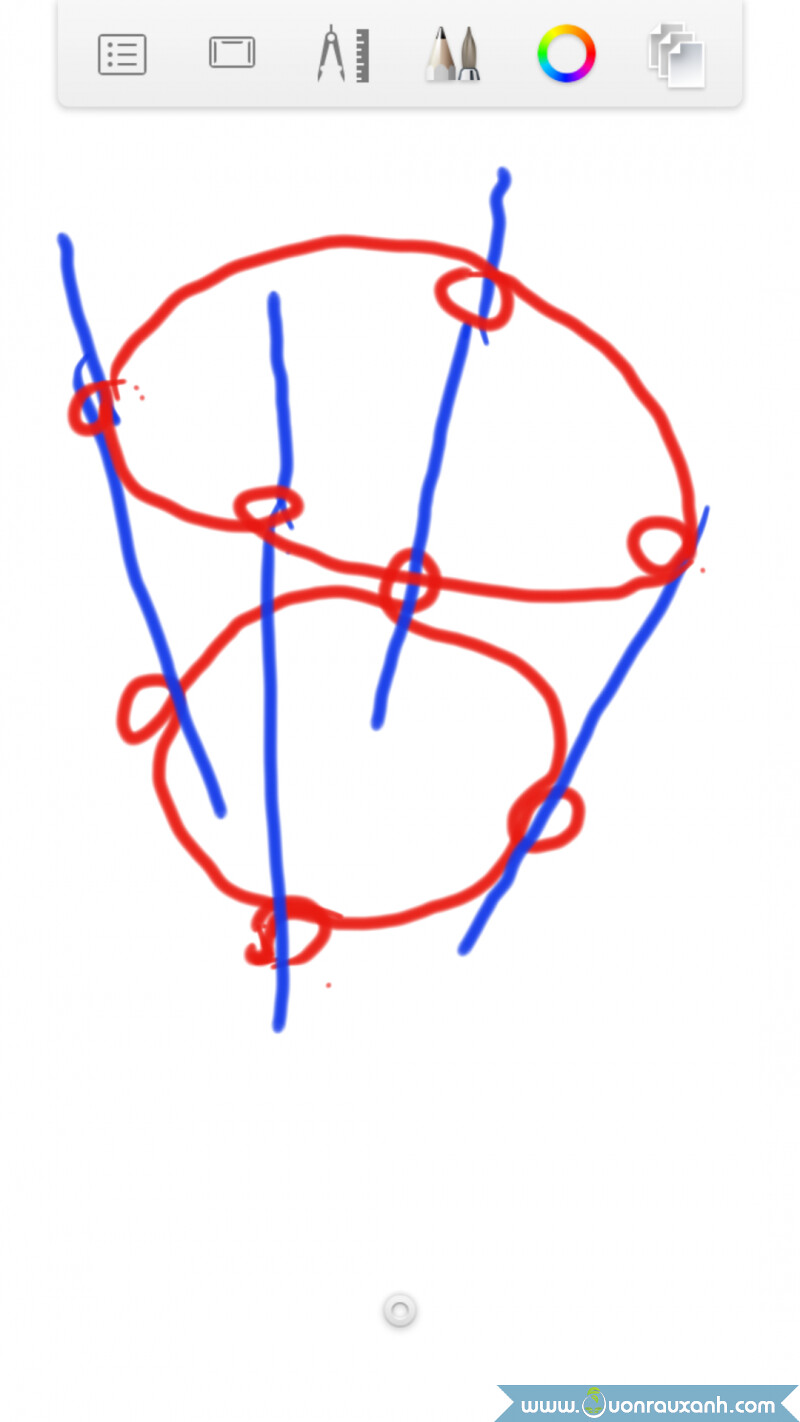This image depicts a digitally drawn illustration created on a touchscreen phone. The artwork features two primary geometrical shapes: a red funnel or cone and a blue sphere. The red funnel and the blue sphere appear connected to each other, forming a striking contrast between the two colors and shapes. The simplistic nature of the drawing highlights the use of vibrant colors and basic forms, creating a visually engaging piece. The red and blue elements stand out distinctly, capturing the viewer's attention through their bright hues and geometric clarity.